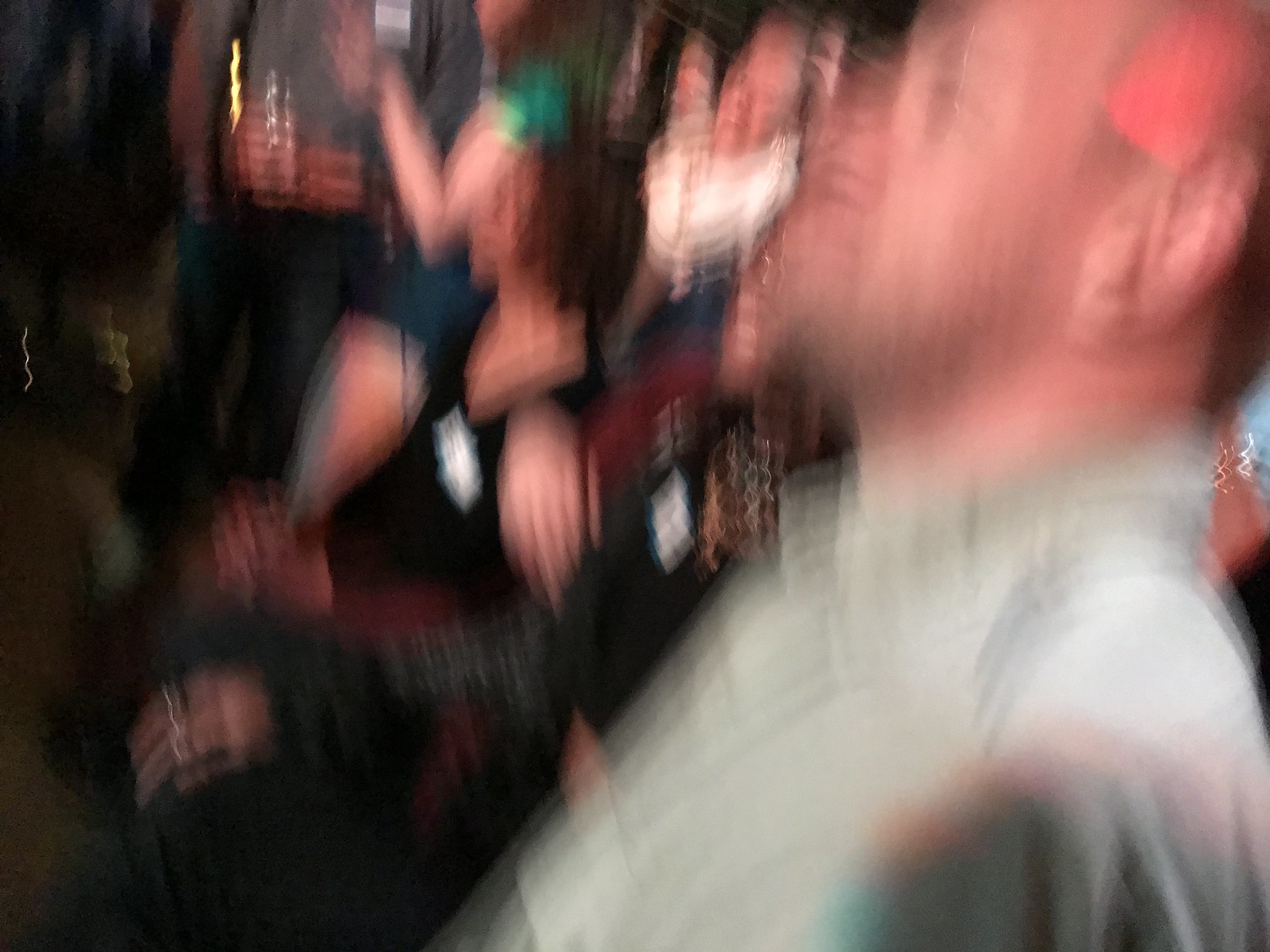This video still captures an indistinct and highly blurred scene, indicative of significant camera motion during the recording. At the forefront is a white-skinned man in profile, wearing a light-colored, collared shirt that might be gray, with a hint of five o'clock shadow on his face. In the background, there emerges the face of an older man with potentially gray hair, seemingly surrounded by a distorted halo of lights due to the image’s severe blur. An arm, bent at the elbow, belonging to another individual in a green short-sleeve shirt is faintly visible, adding to the image's complexity. Amidst the chaos, another indistinct white-skinned hand appears. The entire backdrop is a chaotic blend of vaguely defined human forms, abstract light streaks, and ominous black voids, contributing to the overall disarray and surreal quality of the still.